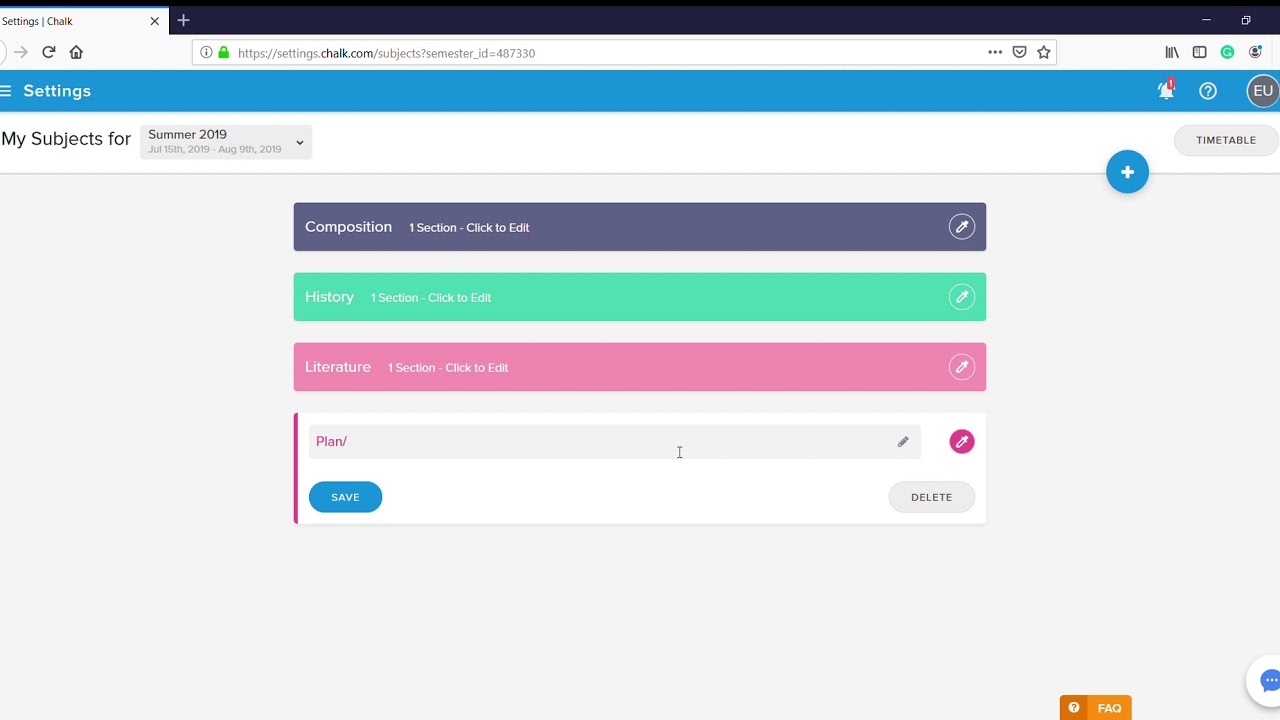A detailed screenshot of an open internet browser is displayed. At the top of the browser, the URL field shows "https://settings.shock.com/subjects?semester_id=487330." The webpage is identified as "Settings Chalk" in black font on the upper left of the browser tab. Just below, there is a horizontal blue bar with "Settings" prominently displayed in white font on the left. On the right side of the blue bar, there is a bell icon with a red notification badge showing the number one, followed by a white circle containing a white question mark. Further to the right, the text "EU" is seen in white within a gray circle outlined in white.

Underneath the blue bar is a white section headed with "My Subjects For" in black font. This heading is followed by a small gray rectangle that reveals a drop-down menu, displaying "Summer 2019: July 15, 2019 to August 9, 2019." On the extreme right side of this section, a gray oval with the word "Timetable" written in black font is visible.